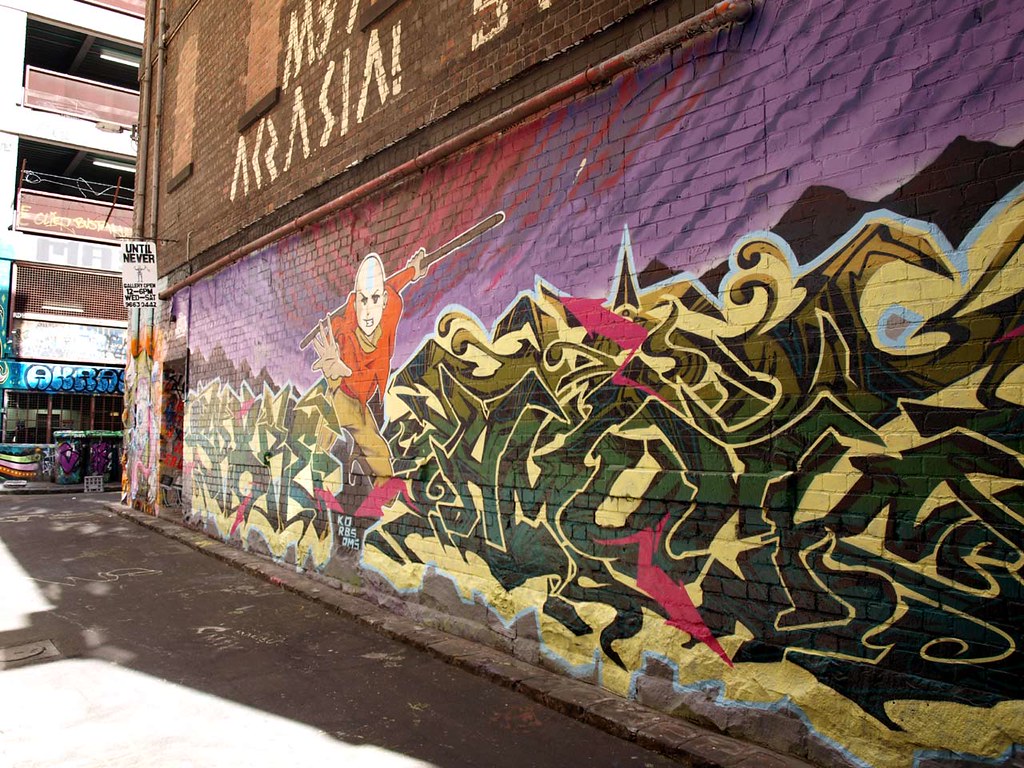In this vibrant photograph, we see an expansive mural adorning the side of a bright exterior brick wall, extending from the right-hand side of the image and shrinking in perspective to the left. The centerpiece of the mural, positioned towards the left of the image, is Aang, the iconic character from the show "Avatar: The Last Airbender." Aang, depicted in a combat-ready stance, is bald and dressed in an orange shirt with light brown pants. He dynamically stretches his right hand towards the viewer while his left hand holds a staff raised behind his back. The mural features bold, graffiti-style lettering in dark green with yellow borders and lines, interspersed with red arrows. This elaborate graffiti, while striking, is difficult to decipher. Above Aang, additional writing also remains unreadable. The mural is surrounded by various urban elements, including a partially visible street and parking lot to the left. In the upper part of the image, there is a street sign that intriguingly states, "Until Never. Gallery open 12 to 6 p.m. Wednesday through Saturday," with a phone number that is not clearly legible. The scene is devoid of people or animals, giving full attention to the dynamic artistry of the mural.